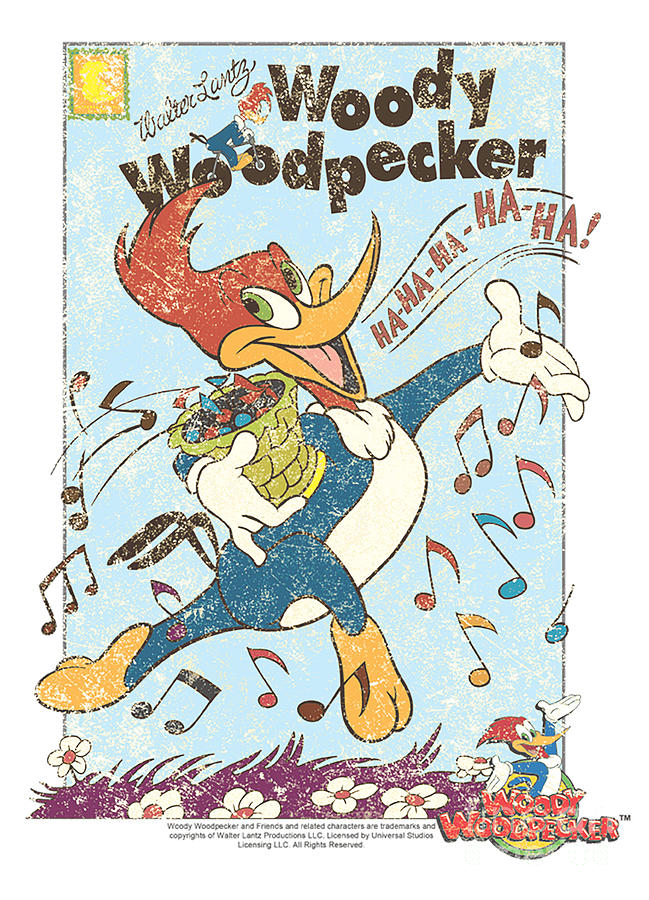This cartoon painting, resembling a page from a book, features Woody Woodpecker prominently. The title "Woody Woodpecker" appears beneath the name "Walter Lanz" written in cursive at the top left. Woody Woodpecker is depicted as a large blue and white bird with a red head, yellow feet, and a curved yellow beak. His striking appearance includes big white eyes with green irises and red feathers that form a crest on his head. 

Woody is joyfully singing, with "ha, ha, ha, ha, ha!" emanating from his mouth in red letters and surrounded by black, red, blue, and yellow musical notes. He holds a green basket in his right hand, filled with red and blue items, and his left hand is stretched out. The scene is alive with motion, as Woody appears to be dancing. 

The bottom of the image shows a maroon patch simulating grassy ground, adorned with white flowers with red centers, and some daisies. Additionally, there is a small Woody Woodpecker figure at the bottom right along with the text "Woody Woodpecker and friends and related characters are trademarks and copyrights of Walter Lanz Productions, LLC. Licensed by Universal Studios Licensing, LLC, all rights reserved."